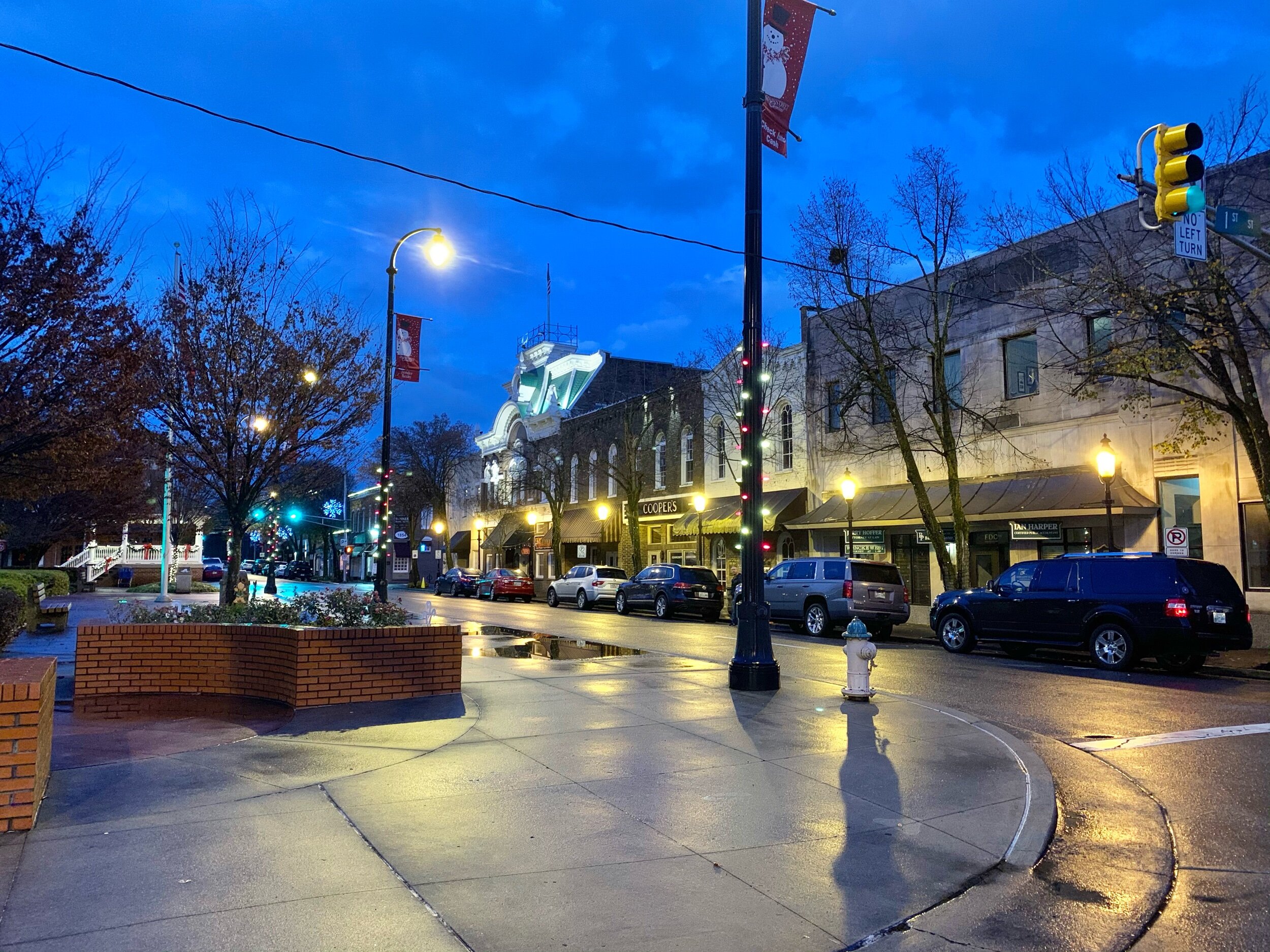The photo depicts a tranquil scene in a small town's downtown area, likely taken during dusk as the sky darkens to a deep blue. Street and decorative lights, including festive Christmas lights, illuminate the area, casting a warm glow over the scene. The town appears quiet and calm, with no movement visible on the empty sidewalks or streets. 

Cars of various colors—black, gray, white, and red—are neatly parked along the sides of the street, in front of connected businesses and down both blocks. These blocks feature a mix of vibrant establishments and residential areas. A green traffic light is visible, adding to the stillness of the moment. 

On one side of the street, small trees, some with orange leaves and some bare, stand in a brick-built median, which also has a floral arrangement. On the opposite side, a white fire hydrant marks a corner where the sidewalk curves around, leading to more businesses and a serene white bridge in the far distance. Adorned poles with snowman flags hint at a festive season. The damp street suggests recent rain, adding a fresh, reflective quality to the scene.